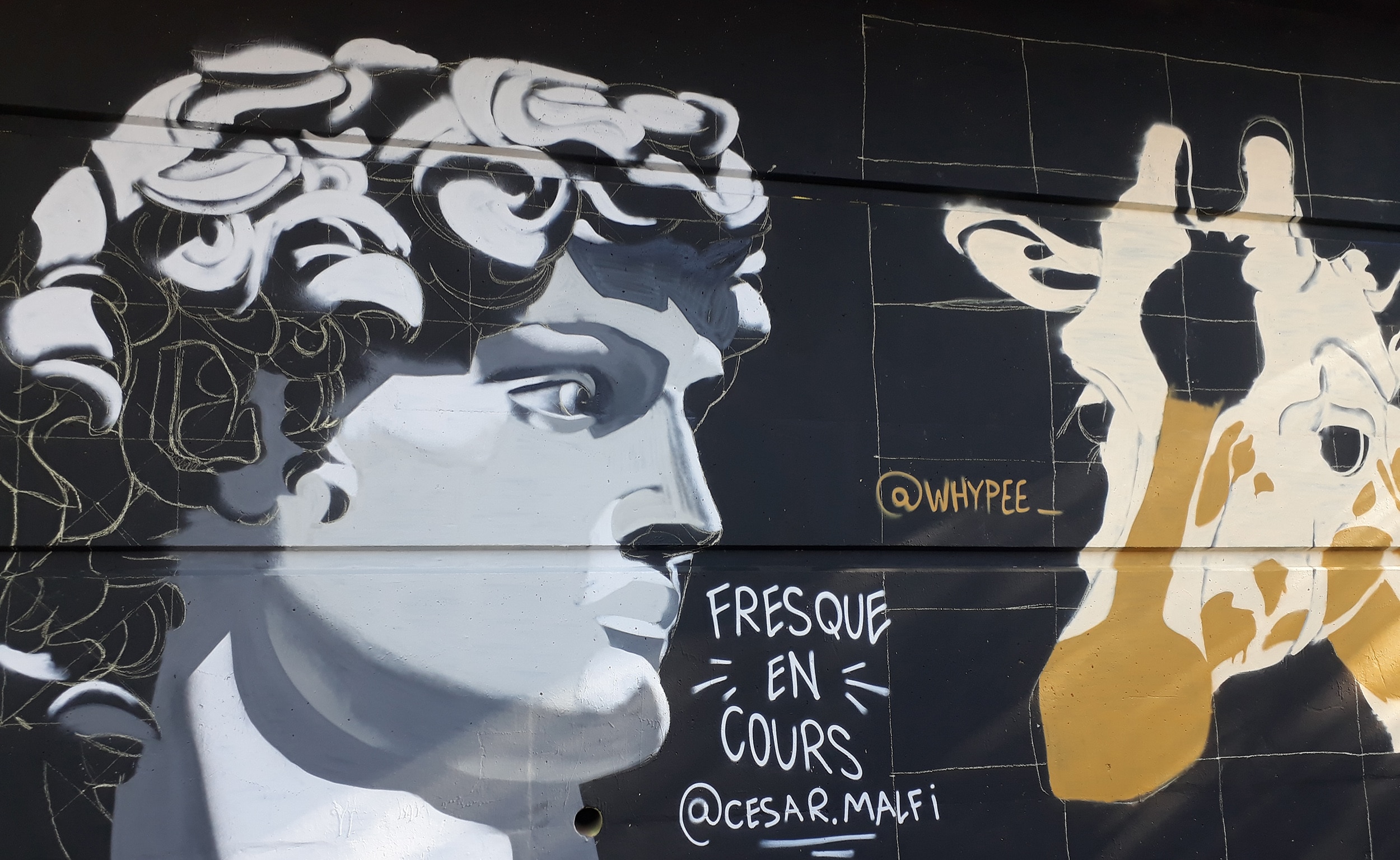The image showcases a striking mural painted on the side of a black building. On the left, there is a highly detailed, 3D-like representation of Michelangelo's David, depicted with curly hair and a realistic, gray-toned face staring to the side. The intricate artistry captures the texture and depth of the sculpture. To the right of David, the word "FRESQUENCOURS" is inscribed in white text, split into three lines: "F-R-E-S-Q-U-E," "E-N," and "C-O-U-R-S." Below this, the social media handle "CESARTMELIFE" is also written in white. Further to the right, a giraffe's head, painted in orange and light tan colors, appears in a conversational stance facing David. Adjacent to the giraffe, the handle "@whypee_" can be seen in brown text. The overall composition stands out against the black wall, creating a visually impactful scene that merges classical art with contemporary street elements.